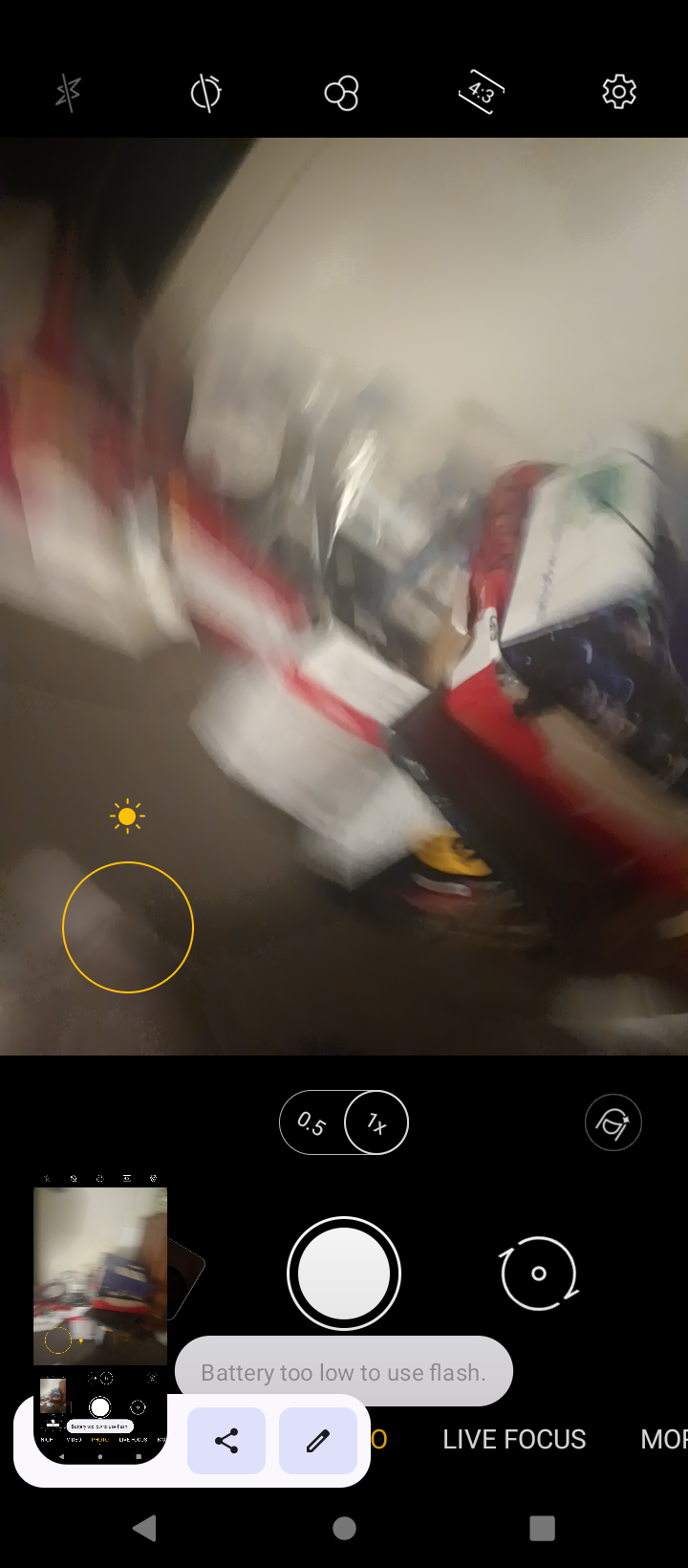In this image, a mobile phone is engaged in photograph mode, capturing a scene that appears blurry and indistinct. The setting resembles a disordered room, scattered with random boxes against a white wall. The phone's screen displays the photography app interface, revealing various settings and notifications. Notably, a message indicates that the battery is too low to enable the flash. The screen also shows a "Live Focus" option at the bottom. Zoom settings are visible, allowing toggling between 0.5x and 1x magnification. A yellow circle signifies the camera's attempt to focus on the subject despite the low battery and cluttered environment.